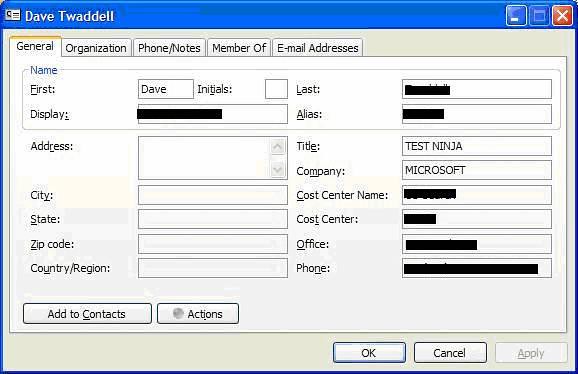This image depicts an older version of a Microsoft contact information window from an operating system such as an older version of Windows. The window features a blue outline at the top, and the title bar displays "Dave Twedell" in white text against the blue background. In the top right corner, the typical minimize, maximize, and red X (close) buttons are visible. 

Multiple tabs are available at the top of the window, labeled as follows: "General", "Organization", "Phone/Notes", "Member of", and "Email Addresses". The "General" tab is currently open. Most of the contact details within this tab have been blacked out, leaving only specific information visible. The entry fields for First Name and Title reveal "Dave" and "Test Ninja", respectively, and the company name "Microsoft" is also visible. 

Additional fields such as Last Name, Display Name, and other details have been obscured with black horizontal lines, likely applied by the person who took the screenshot. At the bottom of the window, there are buttons labeled "Add to Contacts", "Actions", and the confirmation options "OK", "Cancel", and "Apply".